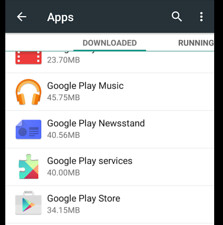This screenshot, captured from an Android cell phone, displays the device's application management menu. At the top left, the word "Apps" is visible alongside a back arrow button to navigate away from this menu. On the top right, there are two options: a magnifying glass icon for searching specific apps, and a vertical three-dot menu for additional settings. 

The menu is divided into two sections: a left column labeled "Downloaded," listing all apps currently installed on the device, and a right column labeled "Running," presumably showing applications that are actively running on the Android device. 

Within the "Downloaded" section, four applications are displayed with their respective sizes:
1. Google Play Music - 45.75 MB
2. Google Play Newsstand - 40.56 MB
3. Google Play Services - 40 MB
4. Google Play Store - 34.15 MB

All listed applications are Google products, emphasizing the prevalence of Google services on the device.